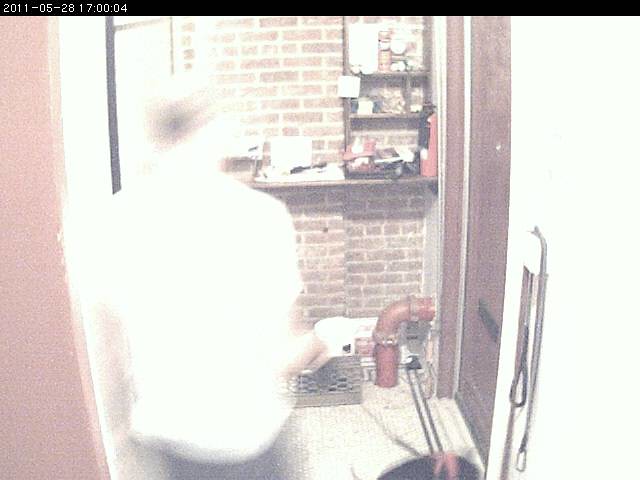This square image, which appears to be slightly overexposed, captures a blurred indoor scene of a basement or utility room, dated 2011-05-28 at 17:00:04, as indicated by a time stamp and black rectangular bar at the top. The left side of the image features a man in a white shirt and dark-colored pants, who is in motion, thereby causing the blur. The background showcases a section of a brick wall and a brick chimney, to the right of which is a brown door or possibly part of a furnace. A prominent red elbowed pipe, which increases in diameter at the base, extends into the floor to the left of the door. Near the chimney's base, a container can be seen holding round objects, adding to the utilitarian setting of the room.